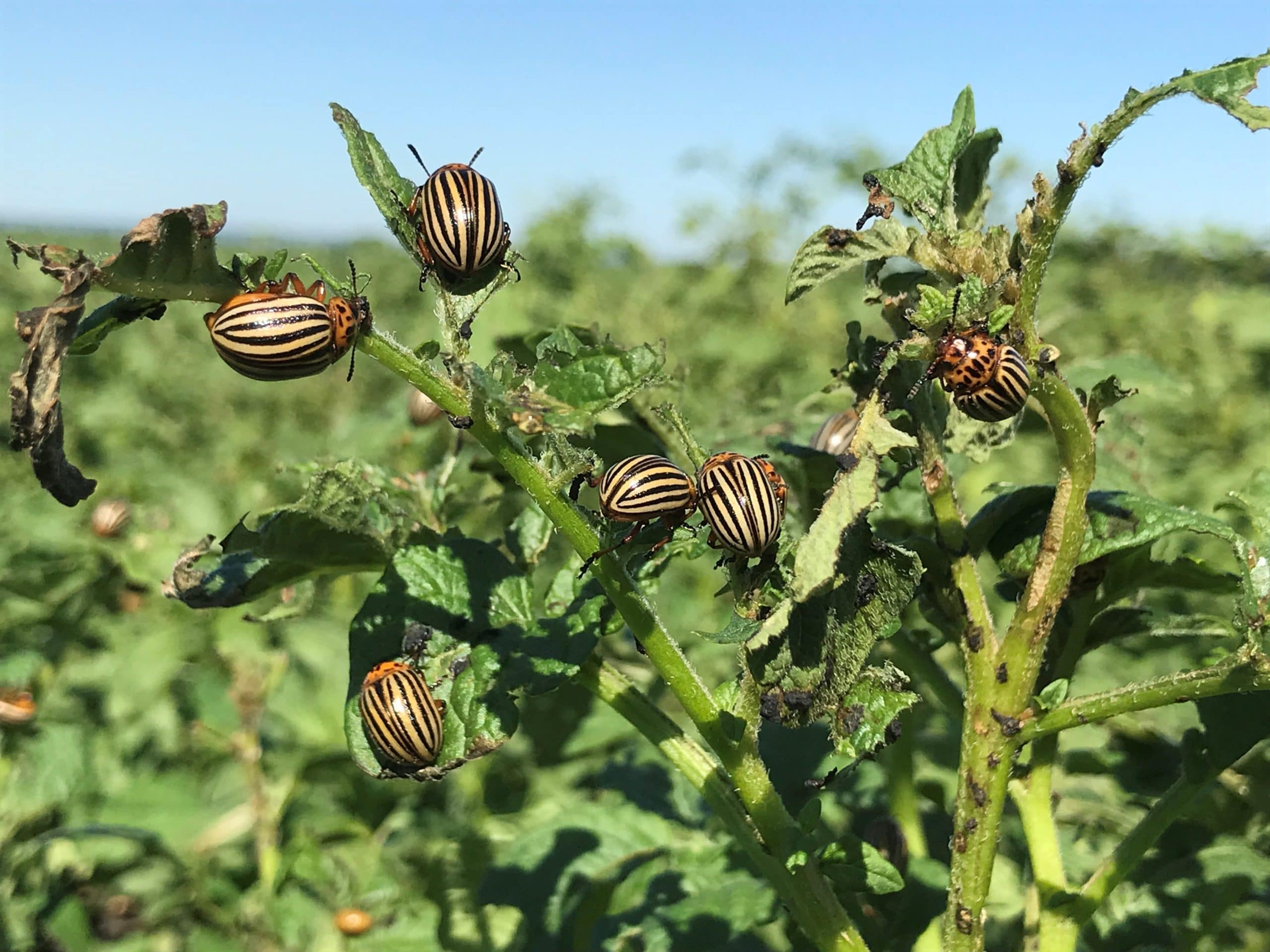In this professionally taken close-up photograph of a green plant, there are six distinct beetles with yellow and black stripes, similar in shape to ladybugs but adorned with strikingly patterned bodies. The beetles are primarily situated on the three main branches of the plant's stems, which are green with both lush and dried-up, browning leaves. The beetles are visibly feeding on the leaves, featuring thin black stripes against broader tan stripes on their bodies, and their heads are orange with varying sizes of black oval spots. Surrounding the focused plant, the out-of-focus background reveals more green plants, hinting at a larger field, with a tree visible at the center and a clear blue sky above, enhancing the natural ambiance of the scene. There is no text overlay, and the predominant colors in the image are neutral greens with accents of dark red from the beetles and a vivid blue sky. This detailed snapshot effectively captures the scene’s essence with a primary focus on the intricate details of the plant and the beetles.